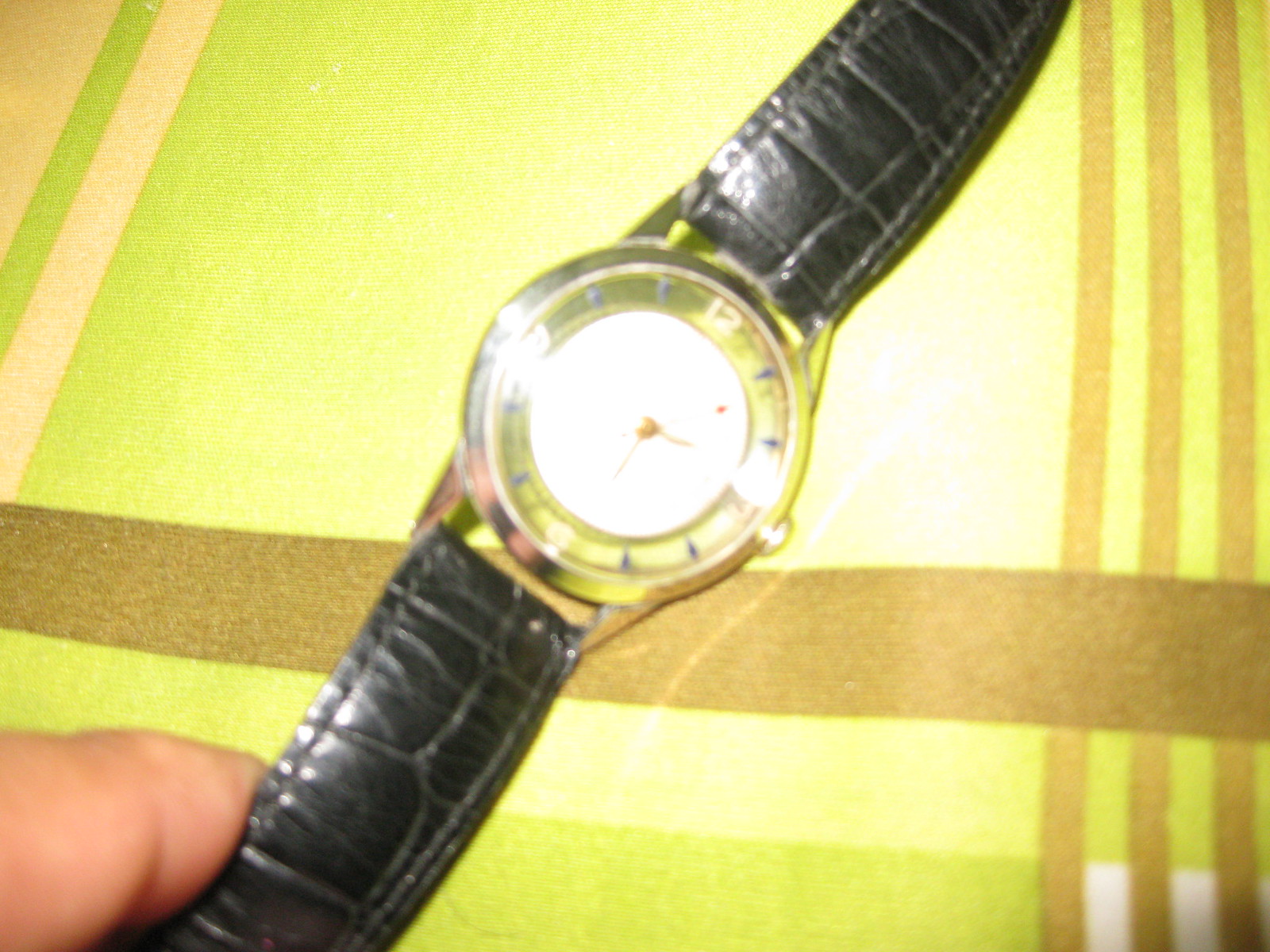This close-up photograph captures a Caucasian hand, likely male due to the thick, muscular finger visible, holding a wristwatch by its black leather strap. The strap enters the frame from the bottom left and the watch extends upward, going off the top of the image. The watch has a traditional circular dial with a white face, prominently featuring the numbers 12, 3, 6, and 9. The remaining hours are marked by blue dashes. The golden hour and minute hands point to a time just before 2:30, with a central golden attachment anchoring them. The background is a checked material, resembling a tablecloth or bedspread, in shades of pea green, brown, and white. The image is quite blurred and suffers from poor lighting, with some areas dazzled by light, which makes certain details harder to discern.